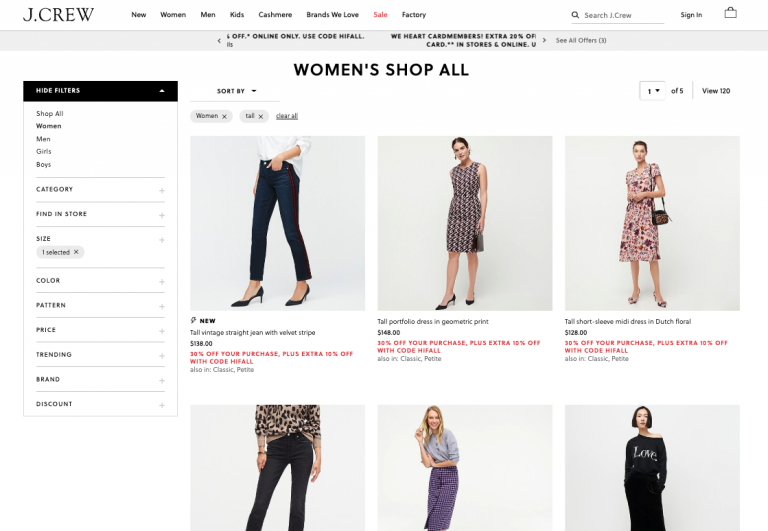The image displays the homepage of the J.Crew fashion retailer's website. The top-left corner prominently features the J.Crew logo. Directly to its right is a navigation bar on a white background offering various menu options, including "New," "Women," "Men," "Kids," "Cashmere," "Brands We Love," "Sale" (highlighted in red), and "Factory." On the far right side of this banner, there are icons for a search function, sign in, and a shopping cart.

Below this, a prominent banner announces special online offers and urges users to apply the discount code "HIGHFALL." To the left side of the main page, there is a sidebar filled with filter options for refining product searches. This sidebar allows users to filter by categories such as "Shop All," "Women," "Men," "Gifts," "Boys," as well as offering dropdown menus for additional options like "Find a Store," specific sizes, colors, patterns, prices, trending items, brands, and discounts.

The bulk of the screen is currently focused on the "Women Shop All" section. It features six high-quality photographs showcasing various women's fashion items. Each photo depicts a different style, ranging from dresses to jeans. Notably, the first photograph has a "New" label beneath it, indicating the freshness of the item in their collection.